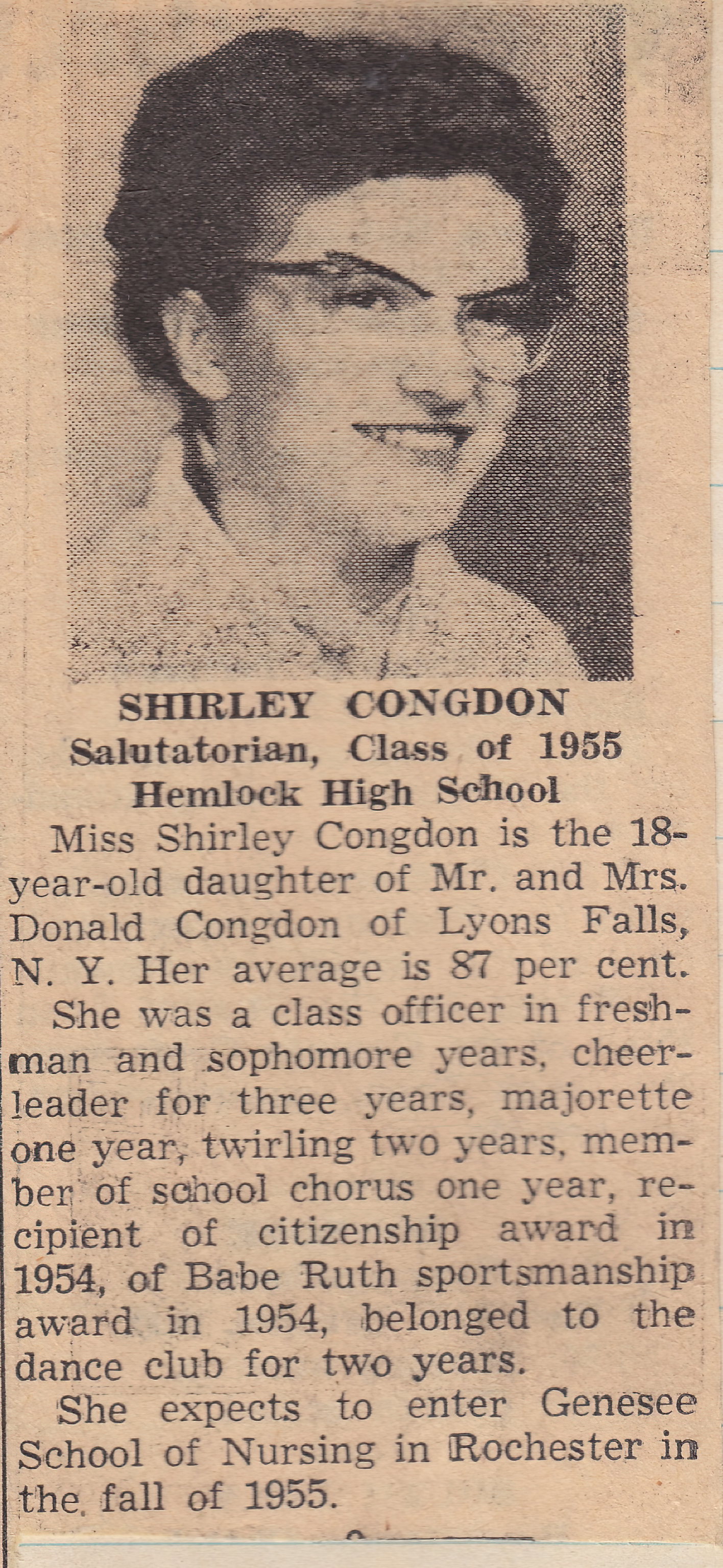This black-and-white newspaper clipping from 1955 features a portrait-oriented image of an 18-year-old Shirley Congdon, Hemlock High School’s Salutatorian for the Class of 1955. The photograph shows Shirley smiling, with dark curly hair and black-rimmed eyeglasses, facing the right side of the image. Underneath the picture, the caption reads: "Shirley Congdon, Salutatorian, Class of 1955, Hemlock High School." The article details that Shirley is the daughter of Mr. and Mrs. Donald Congdon of Lyons Falls, New York, and has maintained an average of 87%. Shirley’s high school achievements include serving as a class officer during her freshman and sophomore years, being a cheerleader for three years, a majorette for one year, twirling for two years, and participating in the school chorus for one year. She was also a recipient of the Citizenship Award and the Babe Ruth Sportsmanship Award in 1954, and she belonged to a dance club for two years. The article notes that Shirley plans to attend Genesee School of Nursing in Rochester in the fall of 1955. The style of the clipping is characteristic of vintage newspapers with black-and-white print.